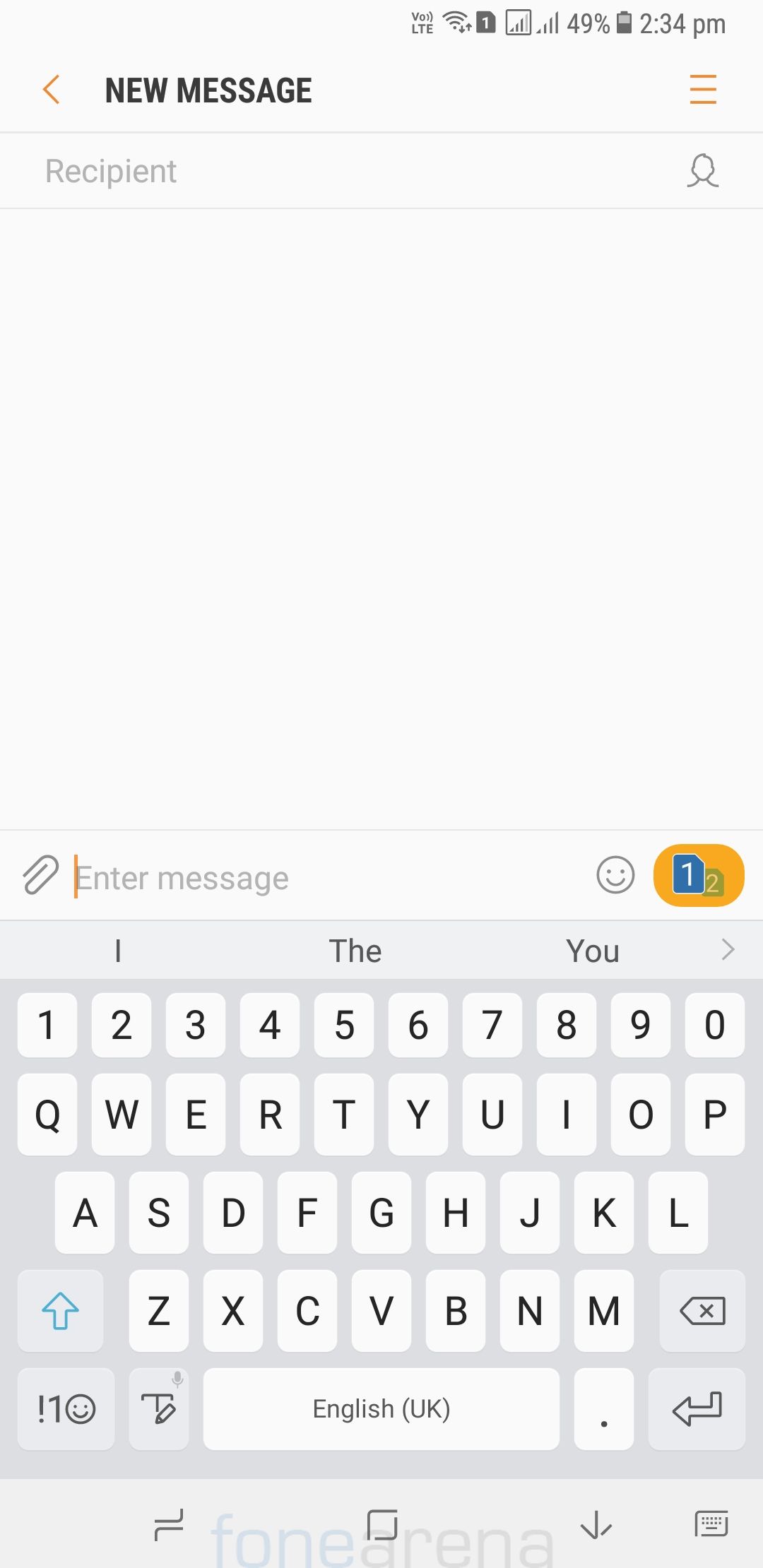The image appears to be a screenshot from a cell phone, presented in either a horizontal or vertical rectangular format typical of such devices. The background is predominantly a white or very light gray hue. In the top right corner, several icons are visible, denoting a 49% battery level and the time as 2:34 PM.

In the upper left section, there is a label reading "New Message," with "Recipient" written in gray beneath it. To the far right of this line is a small icon that appears to represent a person. The central part of the screen is largely blank, characterized by a wide expanse of white, indicating an empty text area.

Approximately halfway down the image, a line divides the screen, followed by a prompt that says "Enter message." A yellow cursor is positioned just before the "E" in "Enter," suggesting that the user is about to type a message. To the right of the text entry space, there is a yellow oval containing the blue number "1" and a smaller green number "2."

Directly below this line is a keyboard layout, ready for the user to input their message.